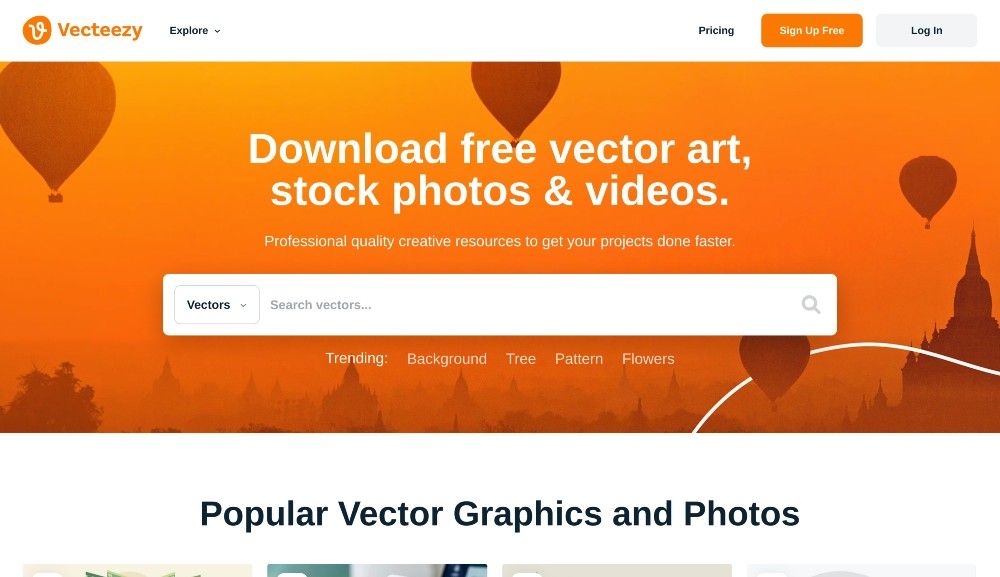Screenshot of the Vecteezy home screen app interface. The top-left corner features the logo "VECTEEZY". Directly to the right is a navigation bar with the options "EXPLORE", "PRICING", an orange button labeled "SIGN UP FREE", and a grey button that says "LOGIN". Centrally located on the screen is a prominent message: "DOWNLOAD FREE VECTOR ART, STOCK PHOTOS, AND VIDEOS", followed by a secondary line of text stating "PROFESSIONAL QUALITY CREATIVE RESOURCES TO GET YOUR PROJECTS DONE FASTER". A search box is prominently displayed in the center of the page, inviting users to begin exploring the available assets.